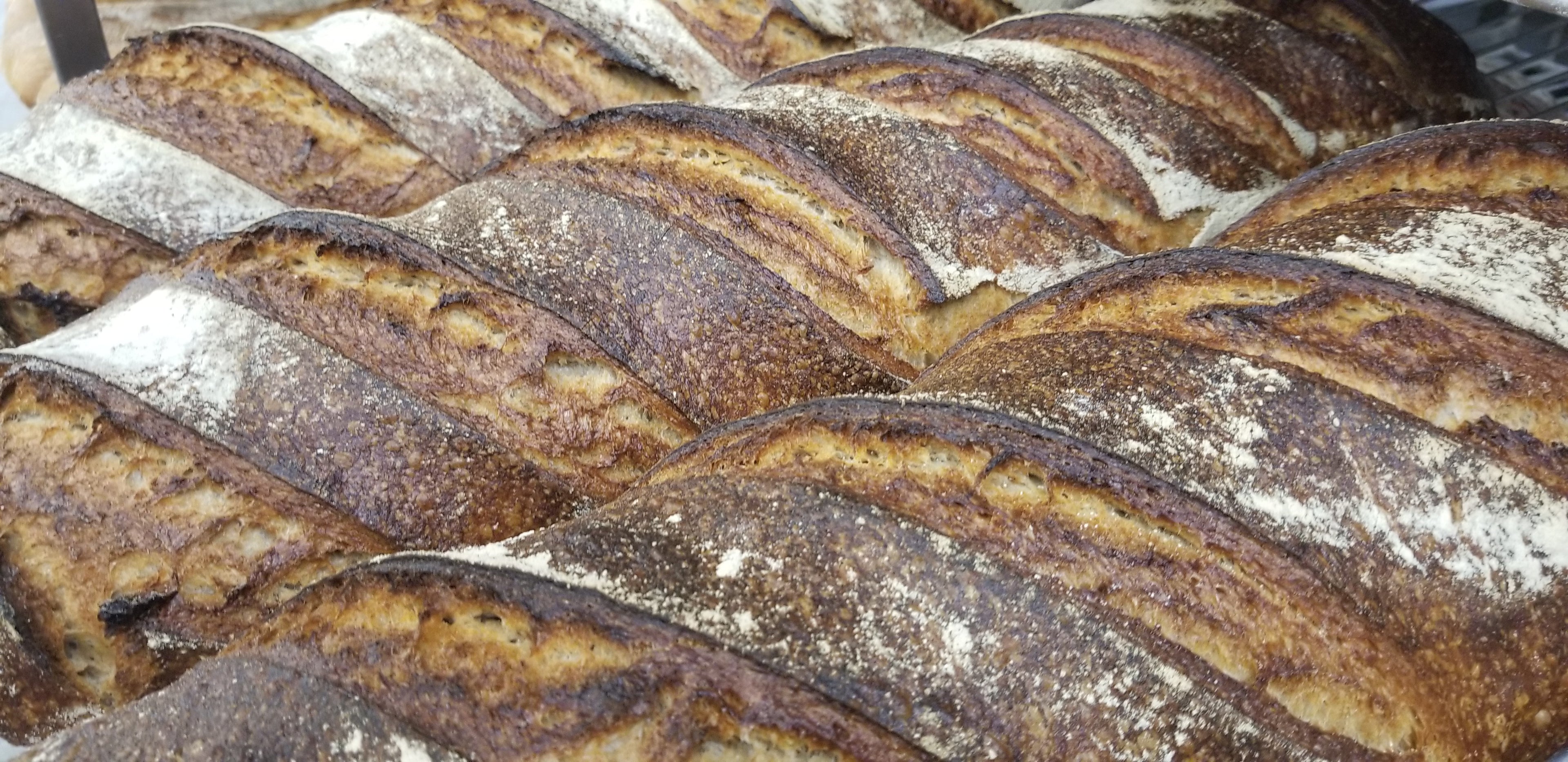This color photo features a very close-up view of three beautifully baked loaves of bread, possibly from a bakery. The loaves, which resemble French baguettes or perhaps Italian bread, are arranged in parallel lines, extending from the lower left corner to the upper right corner of the rectangular image. Each loaf showcases a golden brown crust with parallel, striped cuts that reveal the soft, puffed dough underneath. A light dusting of white all-purpose flour covers parts of the loaves, adding to their rustic appearance. The image focuses closely on the bread, highlighting their golden, well-cooked exterior and the detailed textures formed by the cuts and flour. There are also unexpected features like button-like objects visible in the top right-hand corner of the frame, adding a touch of intrigue to the composition.